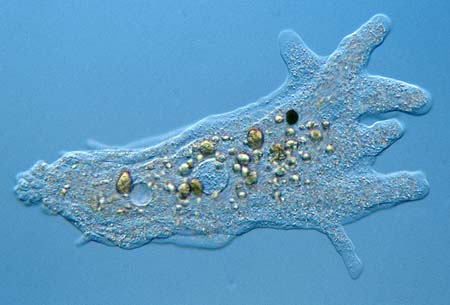This image features a medium sky blue background, reminiscent of a plain piece of paper or canvas. On top of this solid background is a textured, rough material that appears to be spread out like a sprawling, translucent blob, giving the impression of an abstract art piece. This rough, embossed texture seems tactile, inviting touch and exploration. The blob itself resembles sand that has been moistened and allowed to spread, or a goopy substance viewed under a microscope, giving the scene an organic, molecular feel. Toward the upper right-hand corner, the material fans out into several finger-like projections, reminiscent of starfish arms. Embedded within this blob are various pieces of rock and metallic flecks of differing sizes and shapes. These specks range in color from shades of gold, brown, and white to darker browns and blacks. Among these, a particularly large, dark almost-black circle is prominent towards the top center, along with other dense gold and silver pieces that stand out against the more translucent parts of the material. The arrangement of these elements is random, lacking any specific shape, but the detailed textures and contrasting colors make this image a compelling and intricate visual experience.